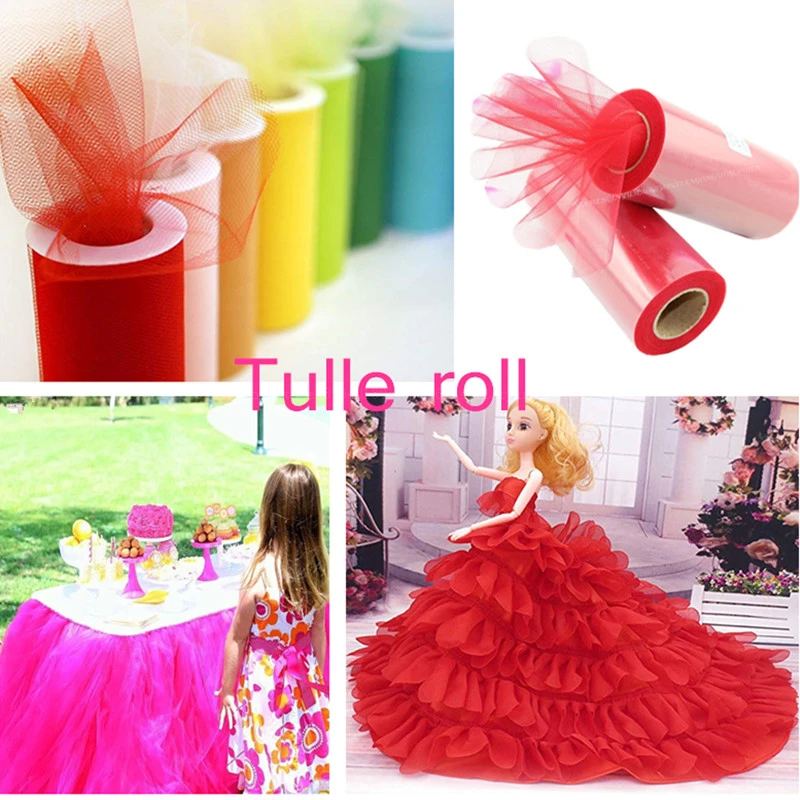The image comprises four separate photographs arranged in a grid, centered around various uses of tulle fabric. The top-left photograph shows several canisters of tulle in vibrant colors like red, white, yellow, green, and blue with some mesh fabric protruding from the tops, suggesting it is tightly wrapped around a cardboard roll. The top-right photo focuses on two canisters of red tulle lying on a white background, providing a closer look at the material's texture. The bottom-left photo features a young girl standing in front of a table adorned with a pink tulle tablecloth. The table, set with cakes and treats, appears to be part of an outdoor celebration, as indicated by the visible grass and floral decorations. The bottom-right photo shows a doll in a dramatic red tulle dress with ruffled layers, standing in a pose as if dancing. Centrally placed pink text reads "Tulle Roll," reinforcing the theme of the advertisement.